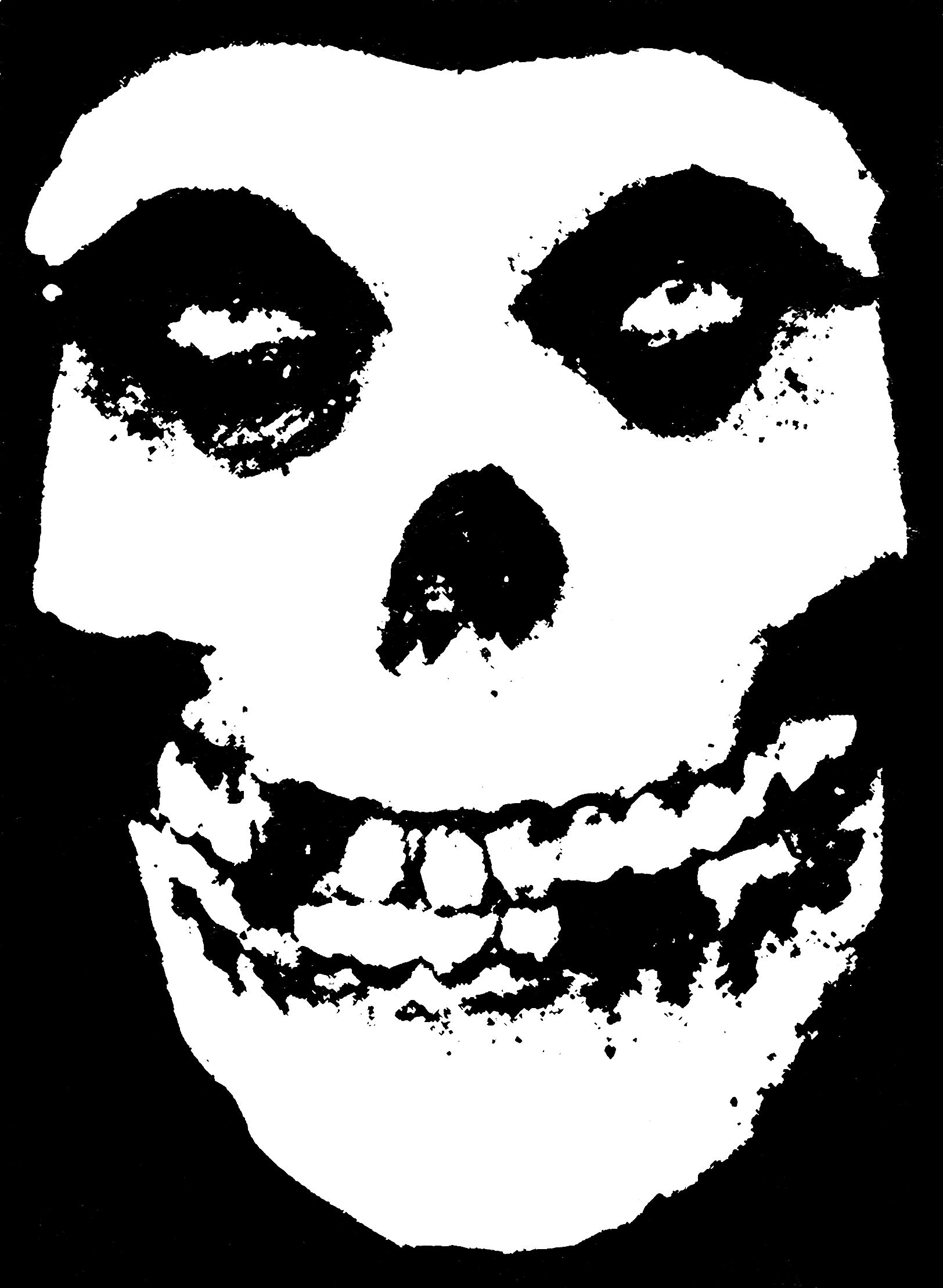This is a detailed black-and-white image of a stylized skull, recognizable as the logo for the punk band, The Misfits. The skull appears cartoonish and grungy, distinctly different from a realistic human skull, with a more monstrous appearance. The white skull features black eye sockets filled with white, blob-like eyes, and a black nasal cavity. Its mouth is partially open, revealing several missing teeth—specifically, there are two gaps on the top row and four or five on the bottom. The top of the skull slopes downward slightly, and the cheekbones are visibly outlined. This iconic image, often seen on T-shirts and novelty items, looks like it was produced using a screen-printing technique, emphasizing the harsh contrast between the white skull and the black background. The stark simplicity and rough edges contribute to its eerie, punk aesthetic, making it a memorable emblem of the band.